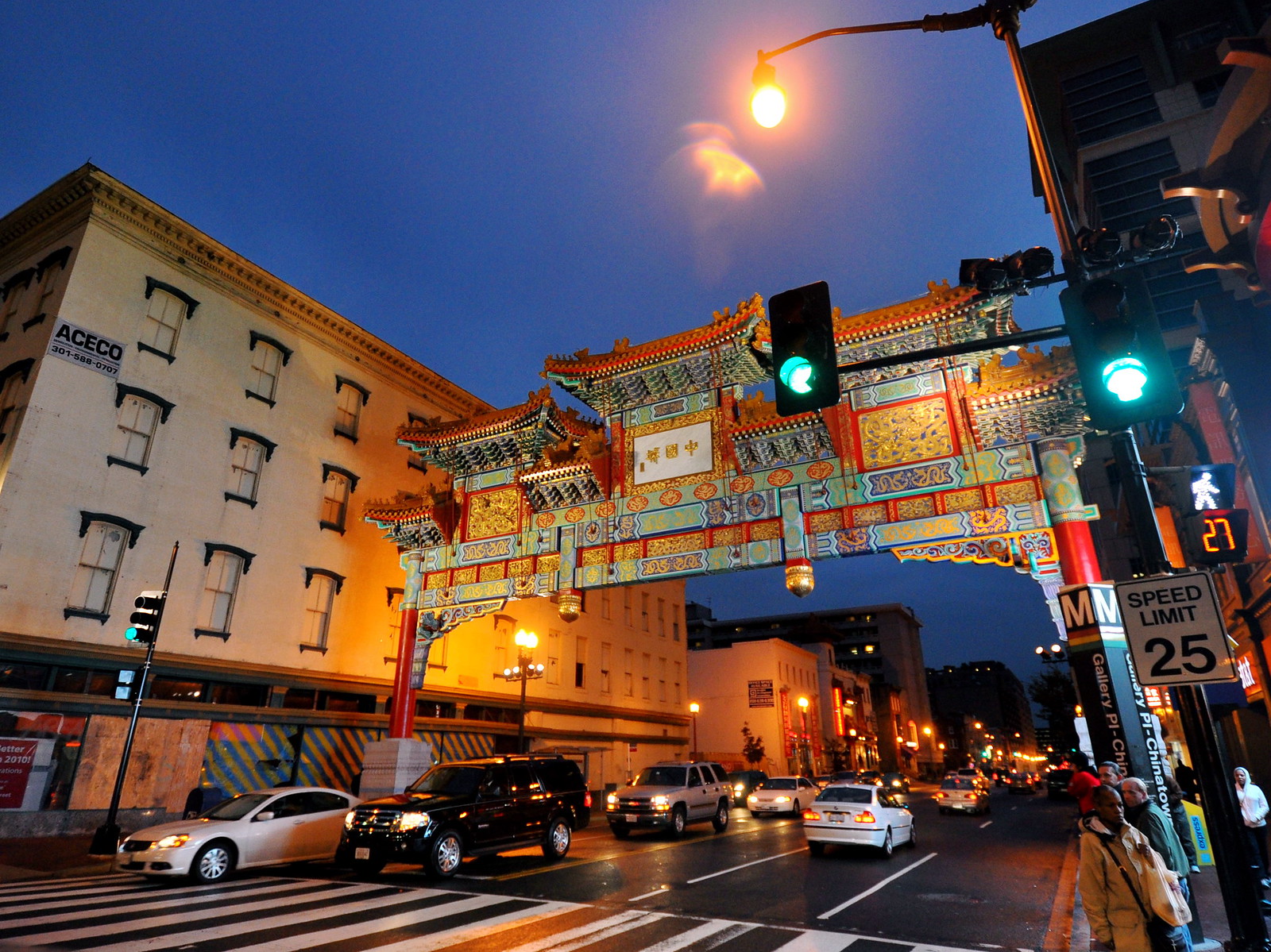The image captures a vibrant downtown scene at the entrance to a Chinatown. Dominating the center is a brightly colored Chinese archway, adorned with intricate dragon details and Chinese symbols in hues of red, gold, blue, and white. This arch, with its distinctive Asian architectural style, spans across a four-lane road bustling with cars. The road, with its polished asphalt, reflects the twilight sky above that is clear with a prominent moon. Flanking the street are city buildings, some modest and unassuming while a notable four-story building on the left appears boarded up, possibly under construction. Streetlights and halogen lights line the sidewalks, casting a glow on the numerous pedestrians. The right side of the image shows a green traffic light and a pedestrian crosswalk sign displaying 27 seconds left, along with a speed limit sign indicating 25 mph. The scene vividly portrays a lively urban area at dusk, highlighting the intersection of traditional Asian culture and modern city life.